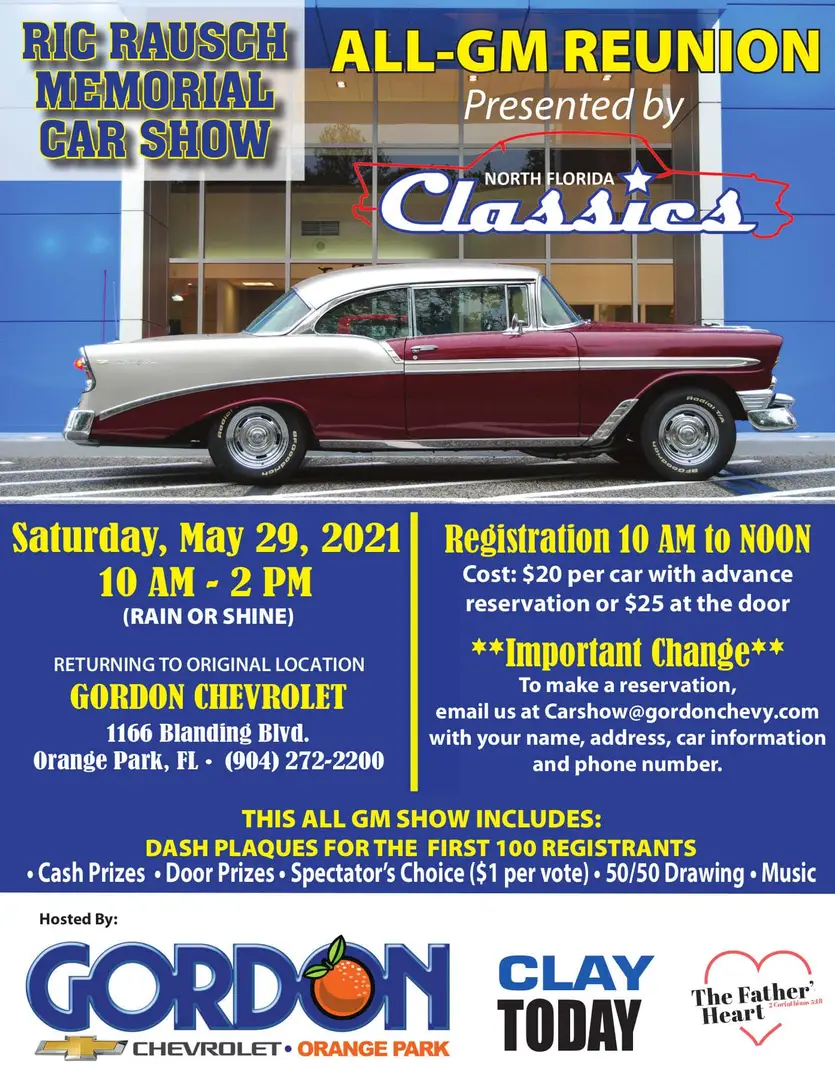The image is an advertisement flyer for the Rick Roush Memorial Car Show, also known as the All GM Reunion, presented by North Florida Classics. The flyer has a colorful design and features a photograph of a classic 1950s-era car, red and beige/cream in color, facing right in front of a blue building with large glass windows.

In bold block text starting at the top left, the flyer announces the Rick Roush Memorial Car Show, slated for Saturday, May 29, 2021, from 10 a.m. to 2 p.m., rain or shine. The event is returning to its original location at Gordon Chevrolet, 1166 Blanding Boulevard, Orange Park, Florida. Contact details include a telephone number, 904-272-2200, and an email address for reservations at carshow@gordonchevy.com, where participants are required to provide their name, address, car information, and phone number. Registration is set from 10 a.m. to noon, with costs at $20 per car with advance reservation or $25 at the door.

Additional information includes perks for attendees, such as dash plaques for the first 100 registrants, cash prizes, door prizes, a spectators’ choice award with $1 per vote, a 50/50 drawing, and music. Sponsors listed at the bottom include Gordon Chevrolet, Clay Today, and The Father's Heart.